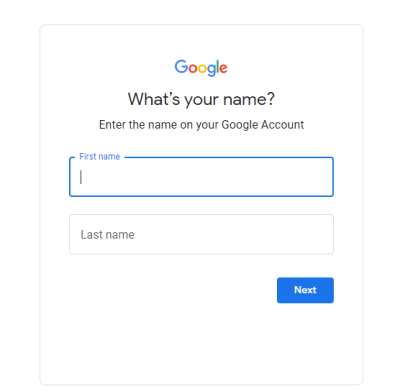The image is a detailed segment of a form from a Google account setup page. It has a larger square with a thin pale gray border encompassing the entire image. 

At the top center of the image, the word "Google" is prominently displayed. The letters are in the distinctive Google colors: the capital 'G' is blue, the first 'o' is red, the second 'o' is yellow, the 'g' is blue again, the 'l' is green, and the 'e' is red.

Below the Google logo, there is a large black text that reads, "What's your name?" followed by a question mark. Underneath this, a smaller instruction reads, "Enter that name on your Google Account," with the 'G' in "Google" and the 'A' in "Account" capitalized.

Further down, there is a blue field encircled by a faint blue outline, labeled "First name" in blue text with a capital 'F'. This field is empty, indicating that the user needs to enter their first name here.

Continuing downwards, another text field appears with the label "Last name" in gray text without any outline. This field is already pre-populated with a last name, unlike the first name field which is blank.

In the bottom right corner, there is a blue rectangular button with the word “Next” centered on it in white text with a capital 'N'.